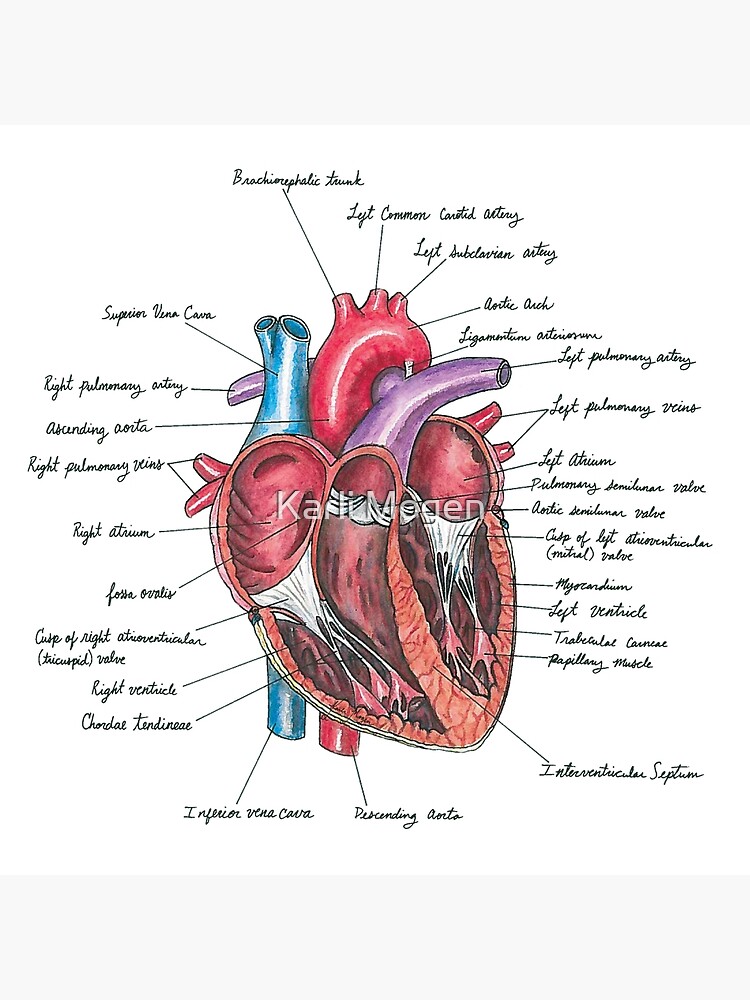The image depicts a detailed cross-sectional diagram of a heart, meticulously labeled with various anatomical features. The heart is shown in vibrant colors, including blue, purple, red, white, and pink, to differentiate between the different parts and chambers. The diagram is centered on a white piece of paper with a thick gray border at the top and bottom. The labels are written in an elegant black cursive script, with arrows pointing to specific parts such as the superior vena cava, right pulmonary artery, ascending aorta, right pulmonary veins, right atrium, right ventricle, brachiocephalic trunk, left common carotid artery, left subclavian artery, aortic arc, fossa ovalis, tricuspid valve, and cauda tendinei. The intricate details and multiple labels, including a central grayish-white label reading "K-A-R-T-I-M-O-G-E-N," provide a comprehensive view of the heart's internal structure and its numerous components.